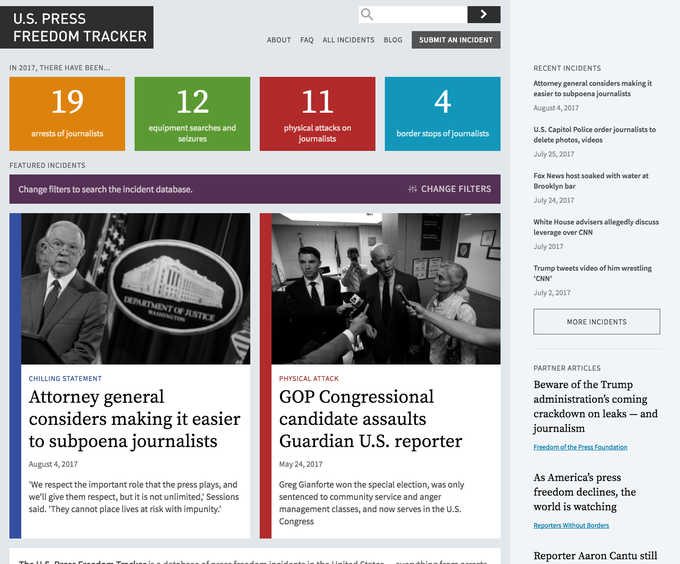This image is a screenshot from the U.S. Press Freedom Tracker website, featuring a predominantly gray background. On the right side, there is a vertical section containing several colored boxes with statistics for the year 2017. A yellowish-orange box displays "19 arrests of journalists," a green box indicates "12 equipment searches and seizures," a red box shows "11 physical attacks on journalists," and a blue box records "4 border stops of journalists." 

Below these statistics, a purple rectangle provides an option to "Change filters to search the incident database," with the text "Change filters" prominently displayed on the right side of the rectangle. 

Further down, a blue rectangle is positioned next to an article titled "Attorney General considers making it easier to subpoena journalists." Above this article is a black-and-white photograph depicting a press conference, likely at the White House or the Department of Justice.

Adjacent to another article, a red vertical rectangle reads "GOP congressional candidate assaults Guardian US reporter." This article includes a black-and-white image showing an individual being interviewed about the incident.